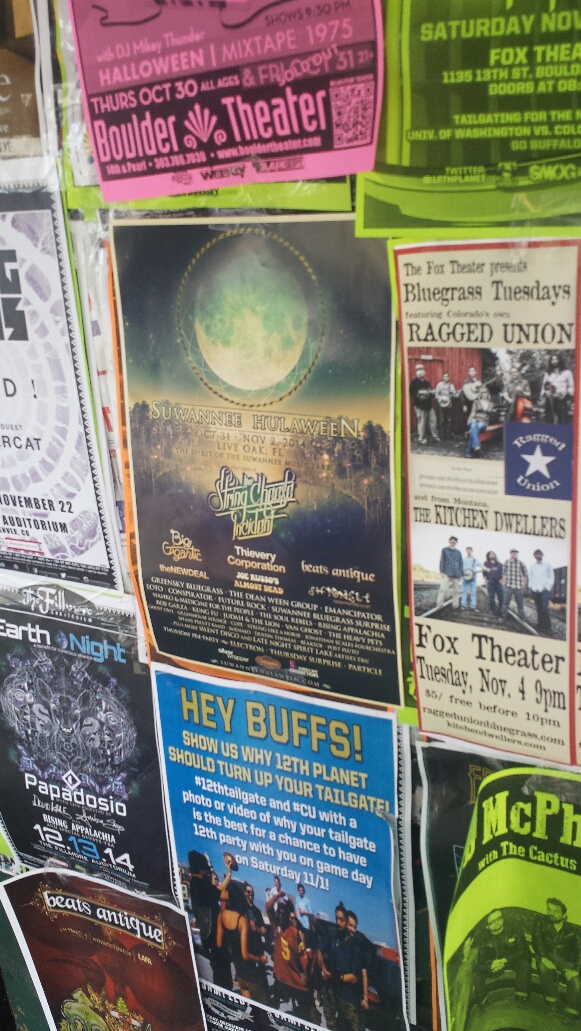This indoor image captures a wall plastered with several event posters, predominantly related to concerts and theater events centered around Boulder. At the top, a striking pink and black poster announces "Halloween Mixtape 1975" at the Boulder Theater on Thursday, October 30th, now sold out. Below it, a central poster features a large picture of a moon with the title "Halloween Antique." Directly underneath, another poster invites University of Colorado (CU) Buffs to showcase why Twelfth Planet should turn up their tailgates, offering a chance for a party on game day, Saturday 11/11. A "Bluegrass Tuesdays" poster is visible to the right, while other posters including "Earth Night" and "Wreckage Union" are scattered around, with some events possibly linked to the Fox Theater, though the exact location varies.